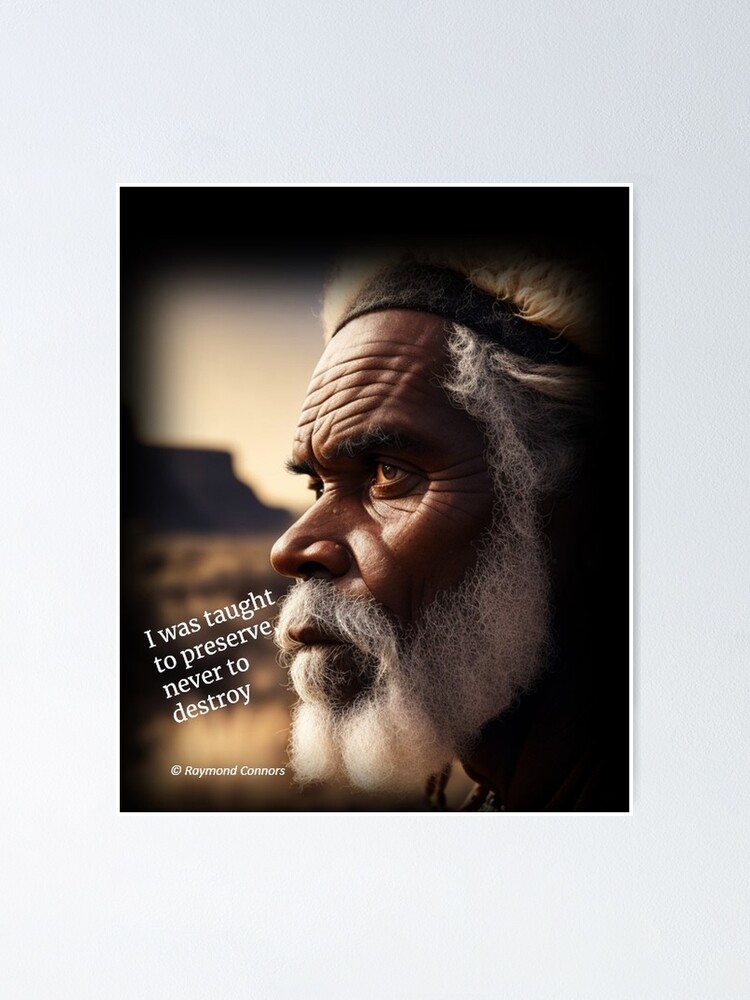This detailed image captures a sepia-toned, close-up shot of an elderly man with a somber expression, gazing off into the distance to the left. The man's face, deeply lined with age, features a very full white beard and white hair, partially covered by a felt headband. His eyes are slightly yellowed, hinting at his advanced years. The blurred background suggests a desert landscape with a small rocky hill, reminiscent of regions like Utah. Diagonally aligned with his beard is the caption, "I was taught to preserve, never to destroy," adding an inspirational and environmental message to the image. A small, indistinct logo at the bottom suggests a copyright by Raymond Connors, indicating the image might be used in an educational or motivational context, possibly as a classroom poster. The overall aesthetic and details evoke a sense of wisdom and a commitment to preservation.